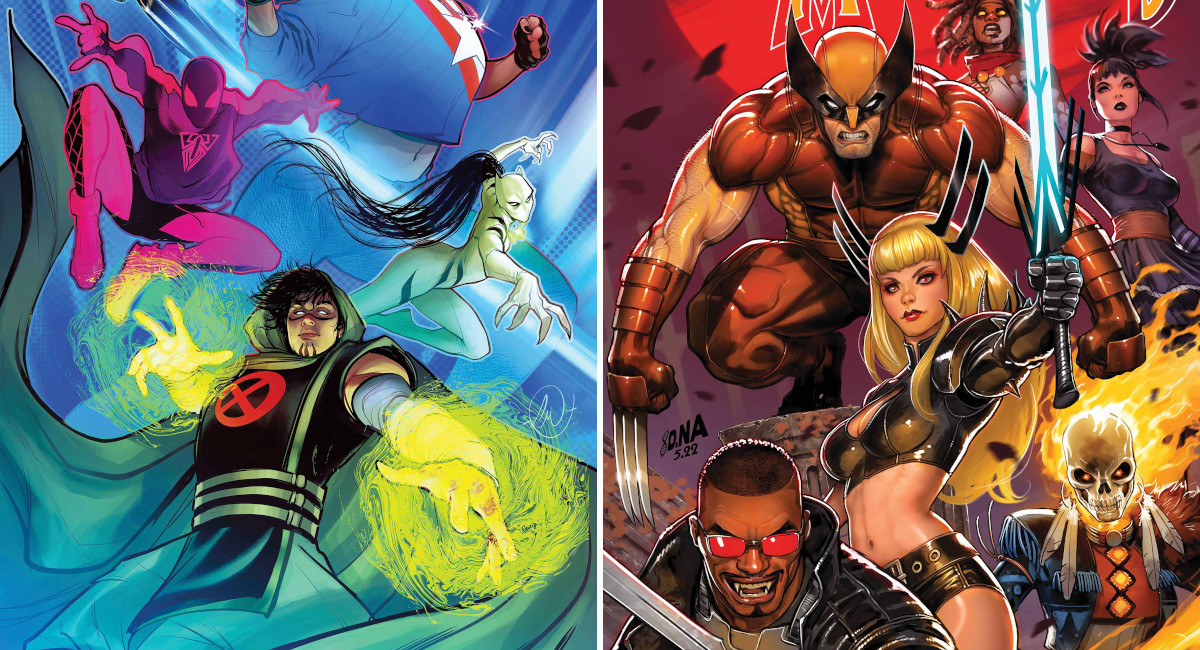The image is a detailed comic book illustration split into two distinct panels. The right-hand side boasts a reddish hue and features iconic X-Men characters. At the center stands Wolverine, brandishing his three sharp claws and clad in red armor, gloves, and pants. Beside him is a fierce woman in a golden-brown bikini, holding a glowing blue sword in her left hand. She has blonde hair and black, spike-like protrusions from her head. Below her, Ghost Rider’s flaming skull blazes menacingly. An African-American man, likely Blade the vampire hunter, is also present, wearing red sunglasses and wielding a sword.

The left-hand side of the image has a bluish-green tint. It showcases characters from the Marvel universe like Spider-Man, who appears jumping into action. In the foreground, a superhero with a red circle and an "X" emblazoned on his black vest has glowing green powers emanating from his hands. Behind him stands a woman with long black hair patterned to resemble cat fur or tiger stripes. Above them, another figure in a blue shirt prominently displays a star on the chest, possibly indicating Captain America. The entire composition teems with dynamic energy and vivid colors, capturing the essence of these powerful comic book heroes.